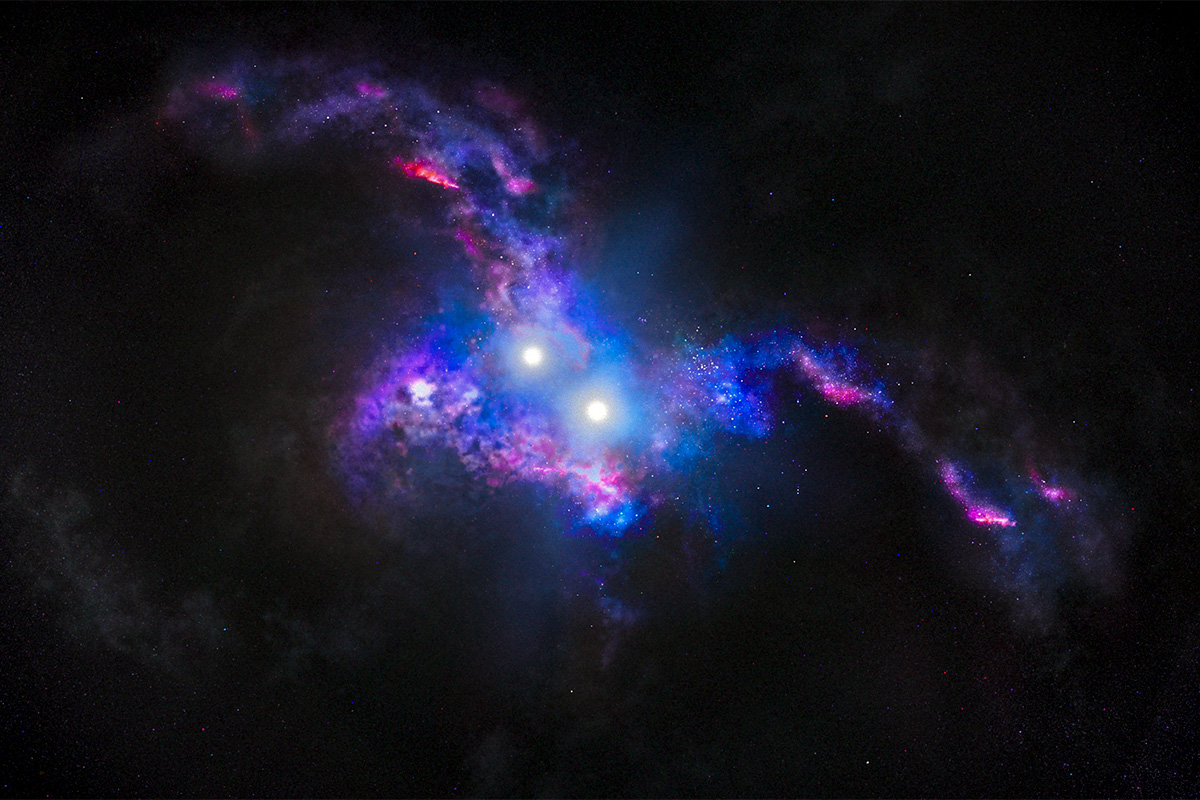The image is a stunning depiction of outer space against a black background, showcasing an array of colorful astral phenomena. Dominating the scene are two bright, circular yellow lights at the center, resembling eyes. These luminous circles are surrounded by swirling hues of pink, blue, and purple, creating an arching, dynamic effect reminiscent of the Milky Way or a nebula. This cosmic display is dotted with countless stars in various colors—whites, pinks, and purples—contributing to the vibrant, magical atmosphere of the night sky. The overall composition suggests a fantastical, almost postcard-like quality, with the colorful patterns extending towards the top left, giving the impression of a bird in flight.